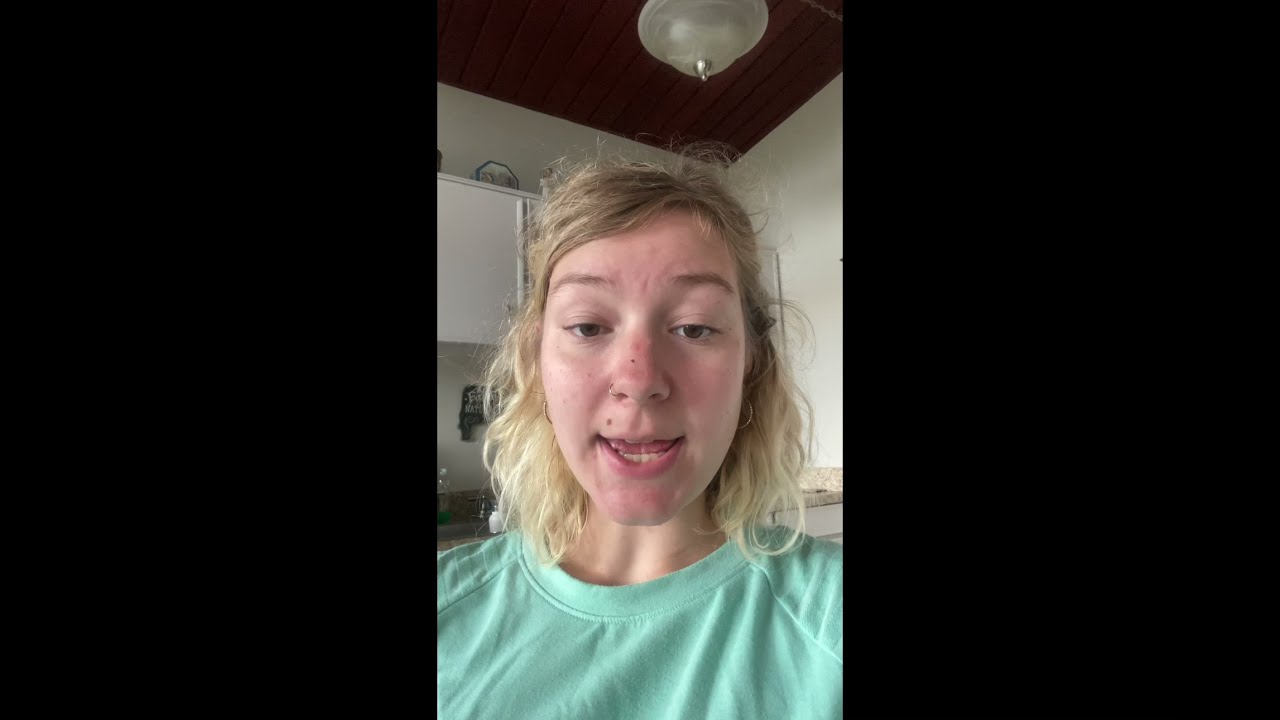The image features a close-up portrait of a young blonde woman, possibly in her late teens to mid-20s, framed in a 9x16 vertical orientation. She is indoors, likely in a kitchen, standing under a circular light fixture hanging from a dark ceiling. The background reveals white walls, wall-mounted cabinets, and what might be a sink, indicating a residential setting. The woman, who has shoulder-length, slightly wavy blonde hair, is wearing a light seafoam green top. Her expression, with eyes open and mouth slightly ajar, suggests she is mid-sentence, possibly recording a video tutorial or vlog. Notable features include a prominent mole between her nose and mouth, pockmarks consistent with acne, earrings, and a nose ring in one nostril. The image appears to be a tight crop, typical of social media platforms like TikTok or Instagram.